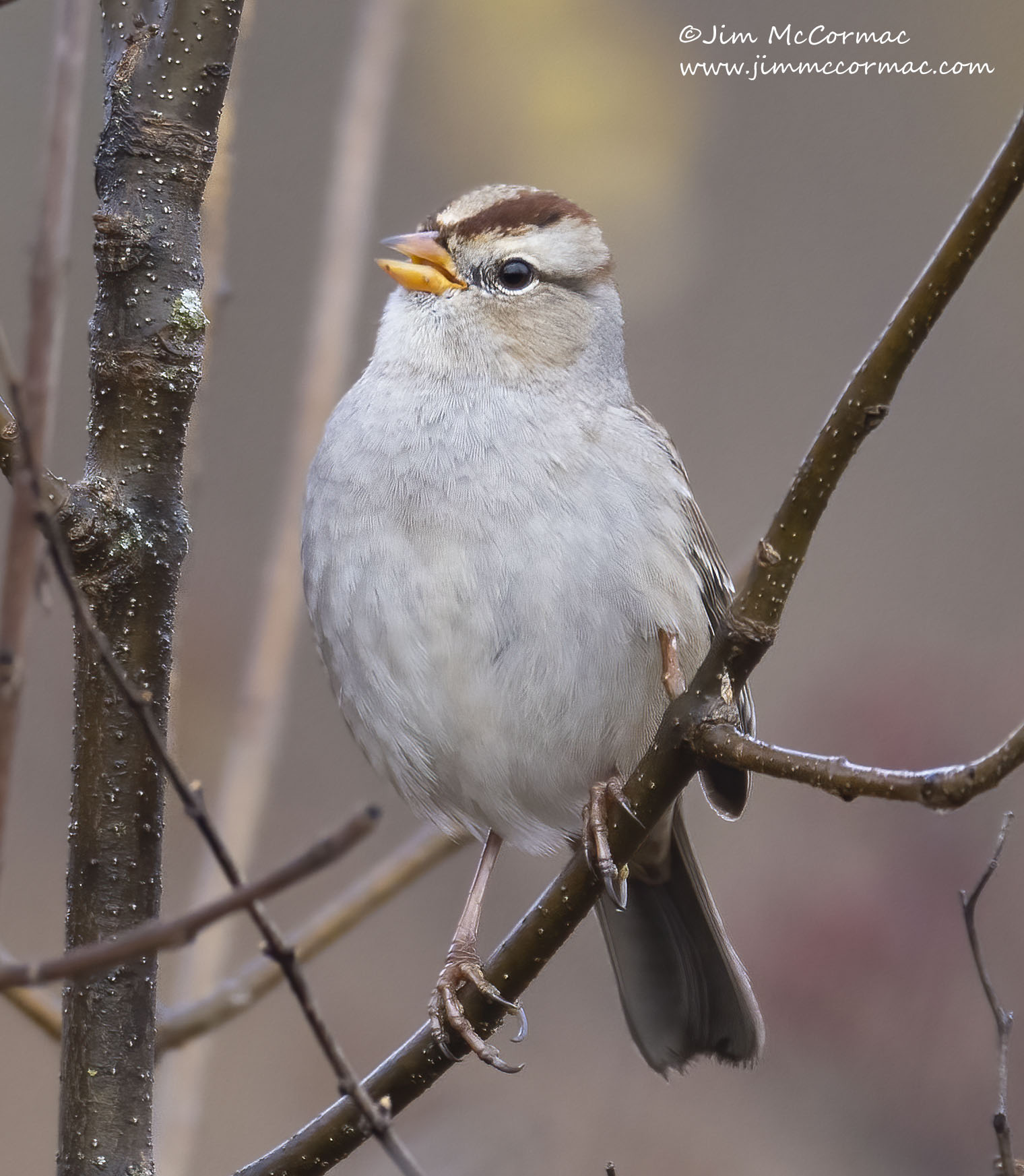The image is a vertically-oriented photograph by Jim McCormack, as indicated by the watermark in the top right corner that reads "@JimMcCormack" with the website "www.jimmcormack.com" beneath it. The photograph, taken outdoors in what appears to be late fall or winter, features a small bird perched on a thin, leafless branch of a tree or bush. The bird, central to the image, has a whitish-gray body with a rounded, squat shape. It displays brown markings on its head, particularly a dark stripe over its left eye with a lighter brown blaze. Its beak is a short, sharp, yellowish-orange with a hint of purple accenting on the top, and it appears to be slightly ajar. The bird's feet are firmly wrapped around the dark brown branch. The background of the image is muted and unfocused, featuring mostly gray tones with subtle hints of yellow at the top and pink in the bottom right area, drawing all attention to the bird as it looks toward the left side of the frame.